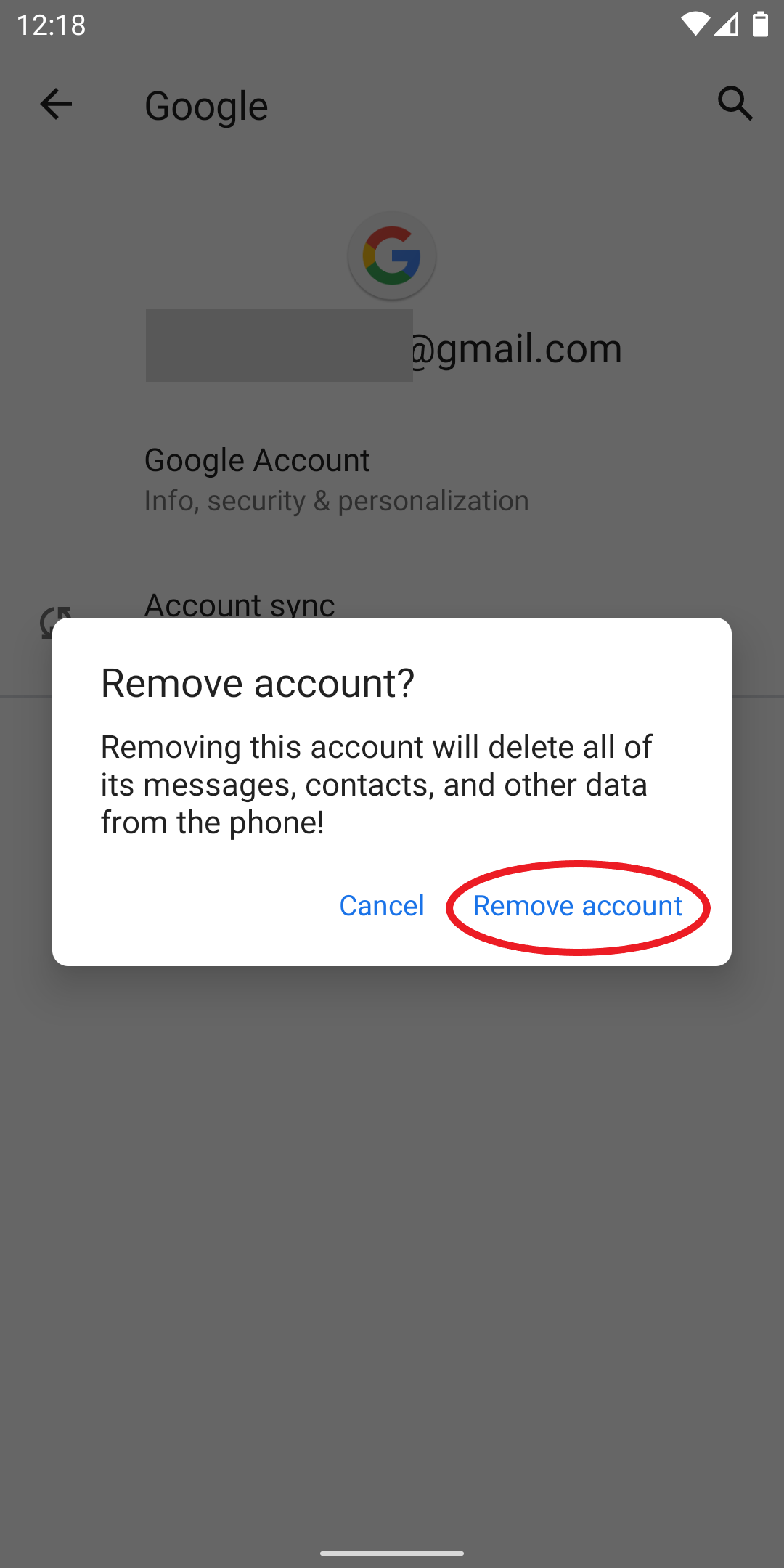This is a high-resolution screenshot captured from a smartphone, set against a slightly hazy white backdrop that appears to have a gray overtone. The centerpiece of the image is a prominent white pop-up box, drawing attention away from the dulled background. Inside the box, bold black text poses the question, "Remove account?" followed by a cautionary message, "Removing this account will delete all of its messages, contacts, and other data from the phone!" Below this warning, there are two actionable options: "Cancel" in blue, slightly to the left, and "Remove account" in blue, accompanied by a small circle with a red bar.

Outside the pop-up box, the smartphone’s status bar is visible at the top. On the left, the time is displayed as "12:18." Moving to the right, icons indicate Wi-Fi strength and phone signal strength, followed by a white battery icon. Beneath this, there is a Google search bar labeled "Google" in black text. Centrally below this search bar, the distinctive Google logo—a circle featuring the colors red, yellow, green, and blue—is displayed. Further down, part of an email address appears; the initial section is obscured by a gray bar, leaving only the "@gmail.com" visible. The text "Google Account" is clearly marked in black underneath the email address. Below this, in gray text, is detailed information on "Info, Security & Personalization," and beneath this, another black header reads "Account sync.” The remainder of the page is obscured by the central pop-up box.